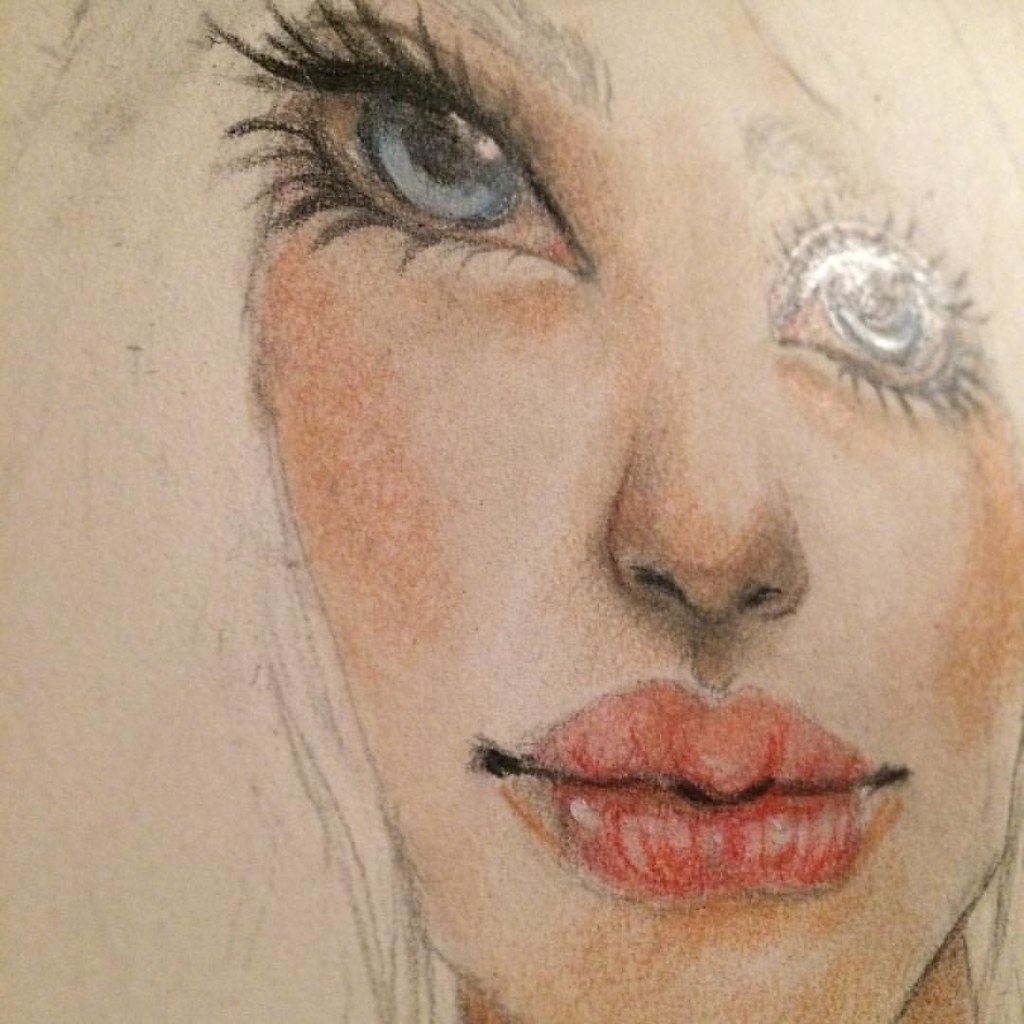This image is a detailed, colored pencil drawing of a woman's face, occupying most of the frame. The woman's face is shaded meticulously with dark and pastel flesh-toned pencils, enhancing her pale skin. She has an intriguing asymmetry in her eyes; her left eye is blue, tilted to the right and facing down, whereas her right eye appears whiter with a partial reflection, set lower than its natural position, and has a rounder shape, creating a disjointed visual effect. Her eyes are lined with long, uneven, and substantial black eyelashes. Her eyebrows are wide and dark, lending a dramatic look to her expression. The woman also has luscious, ample red lips, blending shades of pink and dark red, coupled with a straight, slender nose. Her cheeks show hints of peach and pink, giving them a powdered appearance, as does the tip of her nose. Visible but subtly indicated hair, possibly platinum blonde or uncolored, cascades down the left side while also appearing sketchy on the right. There is a noticeable color bleed around her eyes, making the whites appear red and adding to the striking, surreal quality of the portrait.